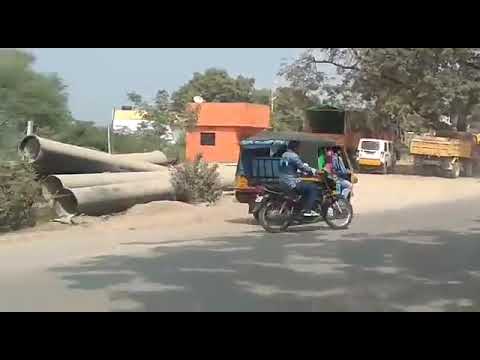In this outdoor daytime image, a man on a motorcycle, wearing a blue shirt and blue jeans, is positioned centrally and riding towards the right. Alongside him, another vehicle heads the same direction. The road beneath them appears to be a regular asphalt road, though some describe it as dirt. Surrounding the road are various elements: to the right, a parking area with large dump trucks and cars; in the center background, an orange building with black windows; and to the left, large pipes, possibly for plumbing, lying next to grassy bushes and some trees. The image, taken in a setting that looks like a developing country, also features small cars and buildings in the distance under a clear, midday sky. The overall color palette includes shades of black, gray, purple, yellow, green, and blue, with no text visible anywhere in the image.